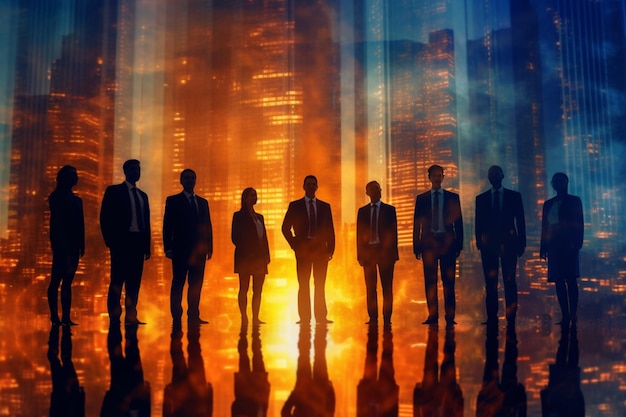The digital artwork depicts a row of nine business people evenly spaced and facing towards the viewer. Among them are three women, positioned at the far left, the fourth from the left, and the far right, distinguished by their business skirts and jackets. The six men are outfitted in black business suits with ties. The figures are mostly silhouetted, with those in the middle slightly clearer, though their feet remain indiscernible. They appear to be standing on a reflective surface, akin to water, which mirrors their images and adds a surreal effect. The backdrop features a cityscape of skyscrapers, partially blurred, with lights in the buildings casting a golden-yellow hue. The central part of the image is dominated by an orange, sun-like glow that tinges everything with a warm, shadowy orange tone. The artwork's rectangular shape is twice as long in width as in height, and the gradient of dark blue in the upper corners adds depth and contrast to the overall composition.